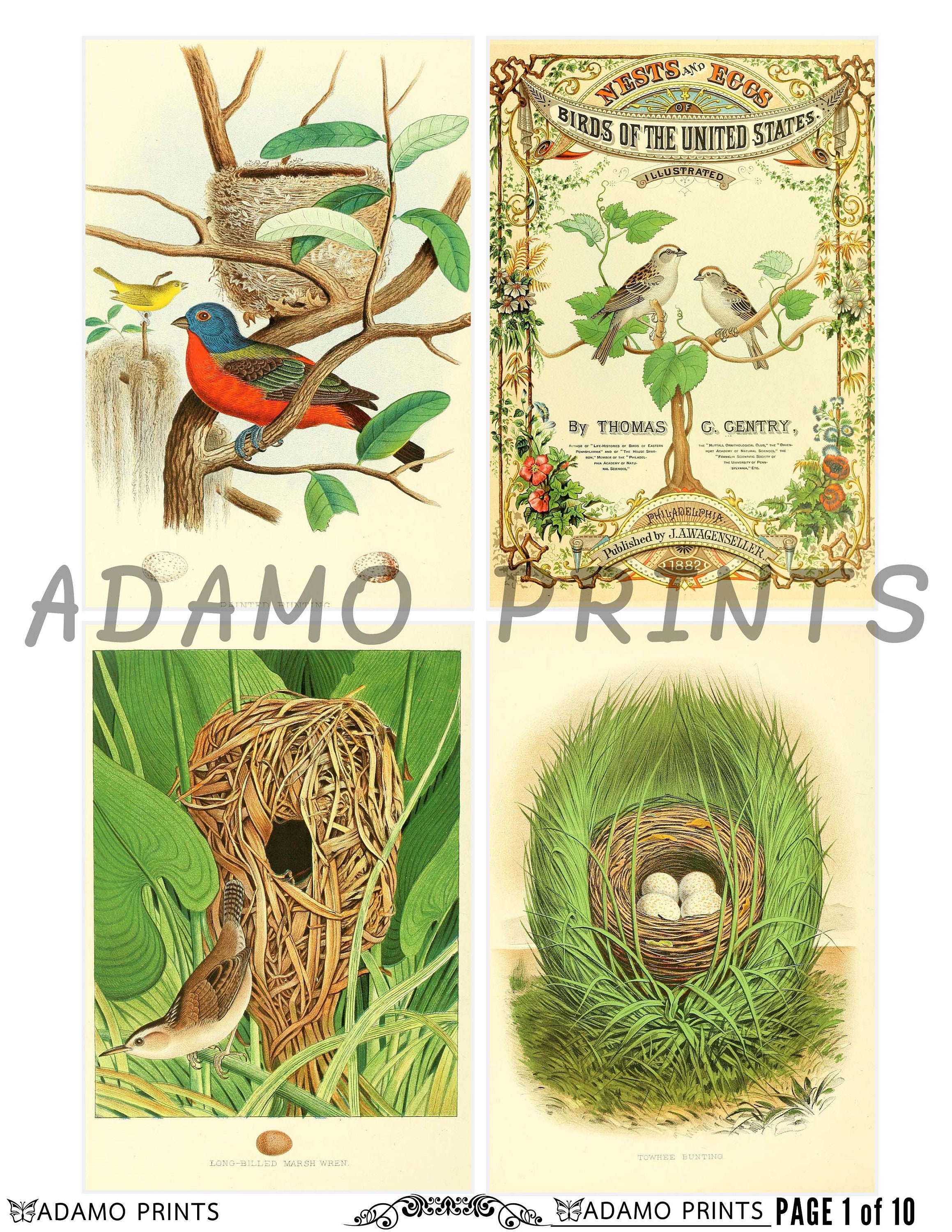The image features a set of four ornithological prints artistically arranged in a collage, with a watermark reading "Adamo Prints" superimposed over the entire composition. In the top left corner, a striking illustration depicts a colorful bird adorned in blue, red, green, and brown hues perched near a nest in a tree, accompanied by a smaller yellow bird in the background. The top right section resembles a vintage book cover or title page titled “Birds of the United States: Nests and Eggs,” by Thomas G. Gentry, adorned with an ornate border of leaves, vines, and flowers. This title page features two birds perched on a tree within its detailed design. The bottom left quadrant portrays a ground nest nestled among leaves and grass, with a brown and white bird resting nearby. Finally, the bottom right image displays a nest cradling four eggs, surrounded by long water reeds and lush vegetation. The watermark "Adamo Prints, page 1 of 10" is subtly positioned at the bottom, adding a branded touch to the natural elegance of the illustrations.